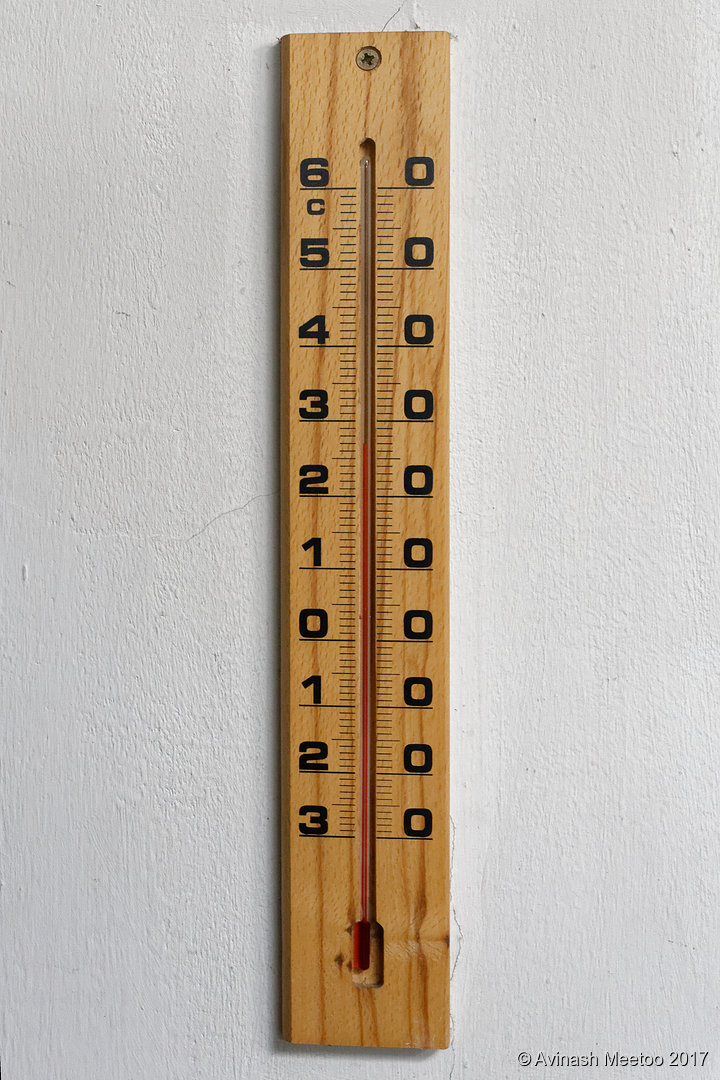This photograph features a meticulously handcrafted vintage thermometer with temperature readings in Celsius. The thermometer showcases an elegant design where numeric indicators are prominently displayed along the entire width of the instrument. The temperature markings begin at 0°C, positioned just below the midpoint, and include 10°C and 20°C, with the zero on the right side of the vertical indicator tube.

The thermometer’s wooden back, which boasts a light maple hue or a finely polished natural wood finish, features striking vertical wood grain patterns that complement the vertical tube. The numeric indicators are large, bold, and easily readable, adding to the functional beauty of the piece. The precision routing for the bulb and tube highlights its handmade craftsmanship.

Mounted on a slightly textured, dove white or dove gray plaster wall, the thermometer is secured with a single flush Phillips head screw at the top. This custom-made, vertically oriented thermometer combines utility and artistry, epitomized in its blonde-colored wood and innovative design that separates the digits along both sides of the tube.